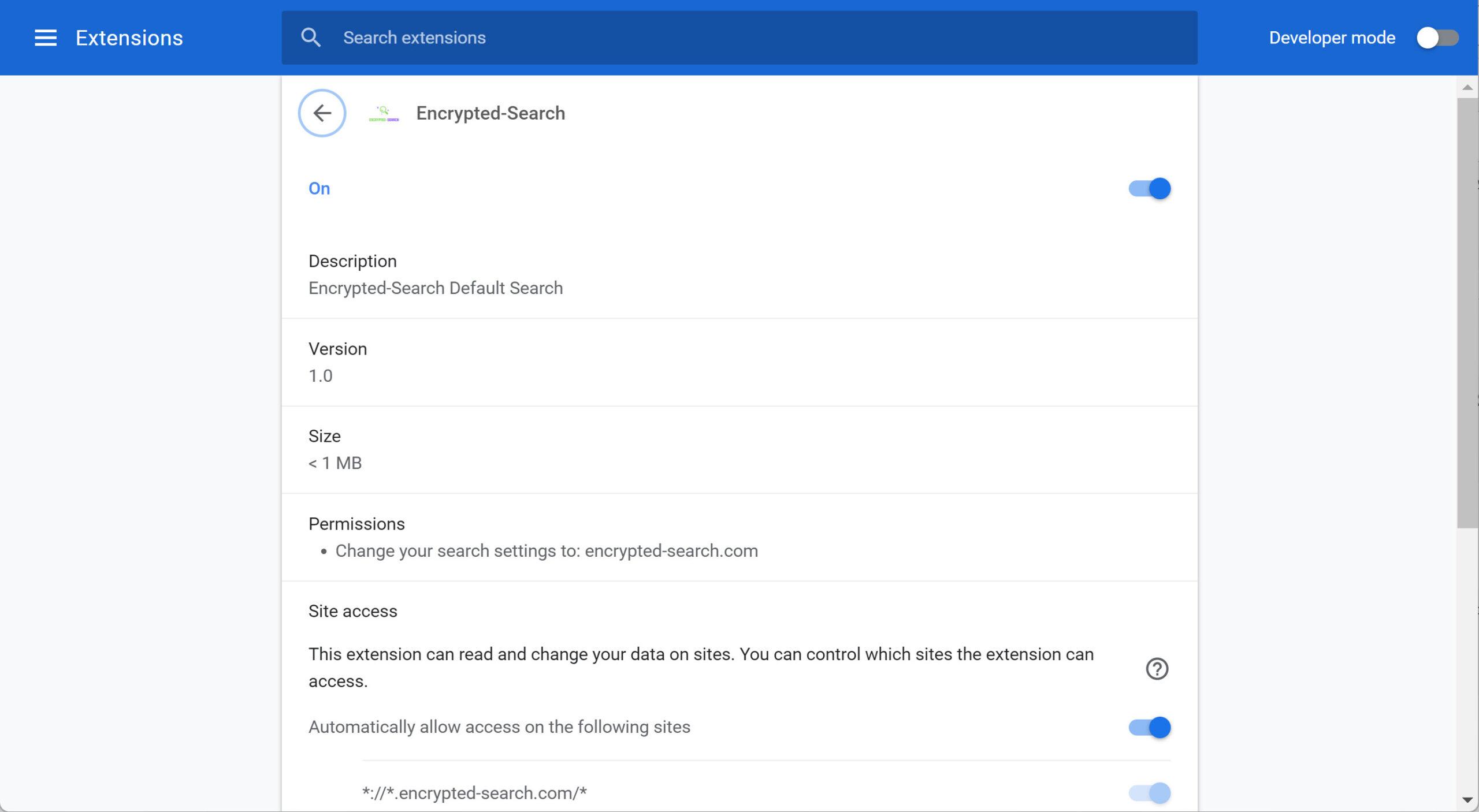Screenshot Caption of a Browser Extensions Page:

The screenshot captures a web browser’s extensions management page. In the upper left-hand corner, the word "Extensions" is prominently displayed. Centrally, at the top of the page, there is a search bar with the placeholder text "Search extensions" typed into it. To the top right, the "Developer mode" option is shown, which is currently disabled, indicated by an unchecked toggle button.

Beneath the top bar, the page displays an extension titled "Encrypted Search." A navigation arrow pointing to the left and a circular motif accompany the extension’s title. To the right of the extension's title, a blue indicator with the word "On" confirms that this option is enabled.

The extension's description follows: "Encrypted Search, default search." Below this, pertinent details are listed:
- **Version**: 1.0
- **Size**: Under 1 megabyte

Permissions for the extension are delineated next, noting that it can change the user’s search settings to utilize encrypted-search.com. There are site access permissions granted to the extension, allowing it to read and change data on sites. Users have control over which sites the extension has access to.

An associated image, a circle with a black question mark inside, is situated next to the following text: "Automatically allow access on the following sites." This option is currently turned on. Below that, a permission rule labeled "asterisk colon slash slash asterisk dot encrypted hyphen search dot com slash asterisk" is shown, with this particular option turned off.